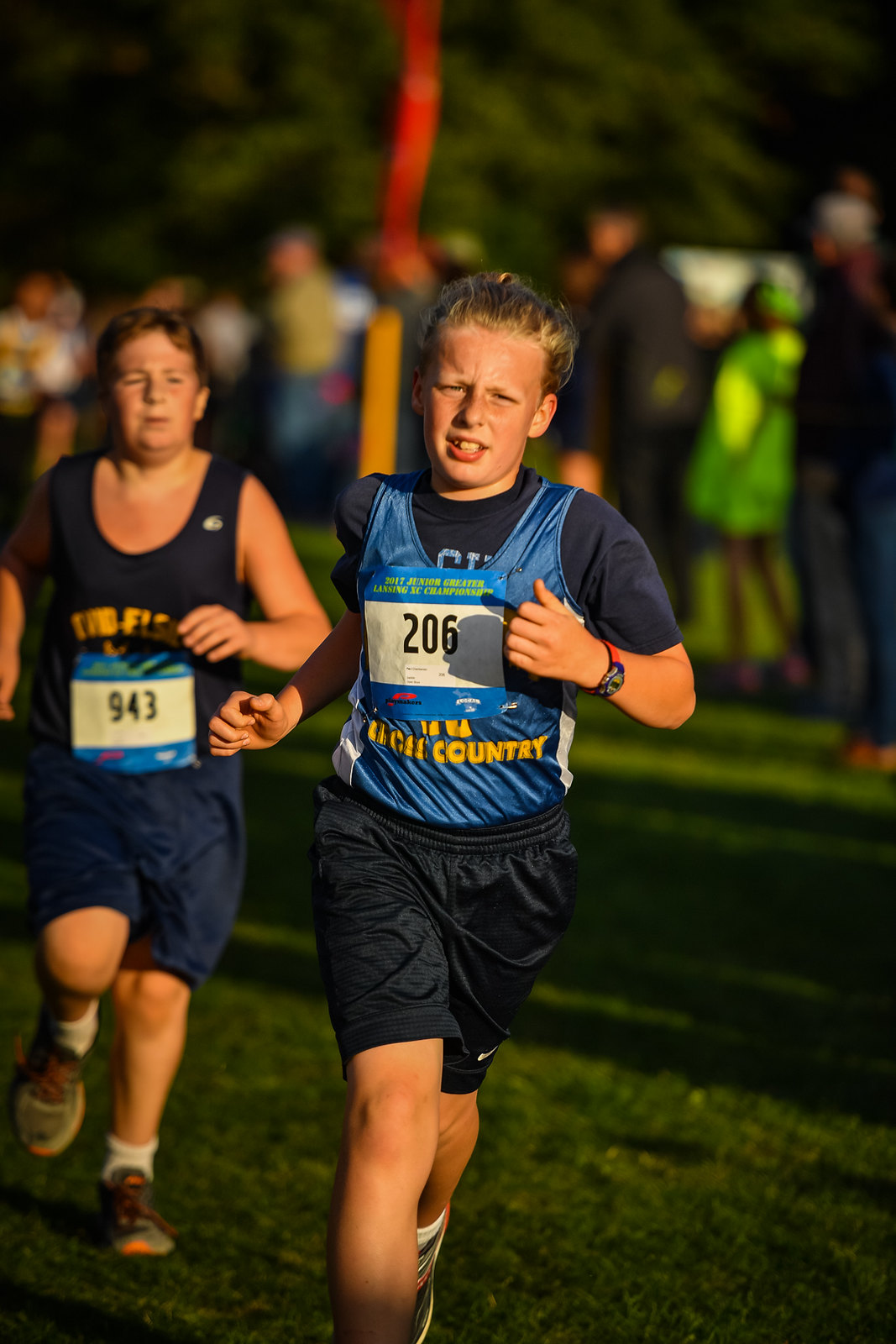The image captures an outdoor scene of two young boy competitors running a race, presumably on a grassy field. Both boys appear to be in their early teens. The boy closer to the camera, with blonde hair, is wearing a blue tank top over a black t-shirt and dark blue shorts, and his contestant number "206" is prominently displayed on a white tag attached to his midsection. His left arm, noticeable by a red-banded watch, is bent at the elbow in a running stance. Slightly behind and to his left, the other boy, who has short brown hair, is wearing a black tank top with dark colored shorts, also to just above the knee, and a white tag displaying the number "943" on his midsection. Both boys are sporting running shoes and sprinting energetically on the grassy terrain, their legs visible down to their shins. The grassy ground beneath them is lush and green, further enhanced by the sunlight which casts long shadows, suggesting a bright and sunny day. In the blurred background, a crowd of spectators, possibly parents or other race onlookers, lines the sides of the field. The backdrop also features out-of-focus trees, adding a sense of depth to the outdoor setting. The entire scene is slightly tilted clockwise, adding a dynamic feel to the photograph.